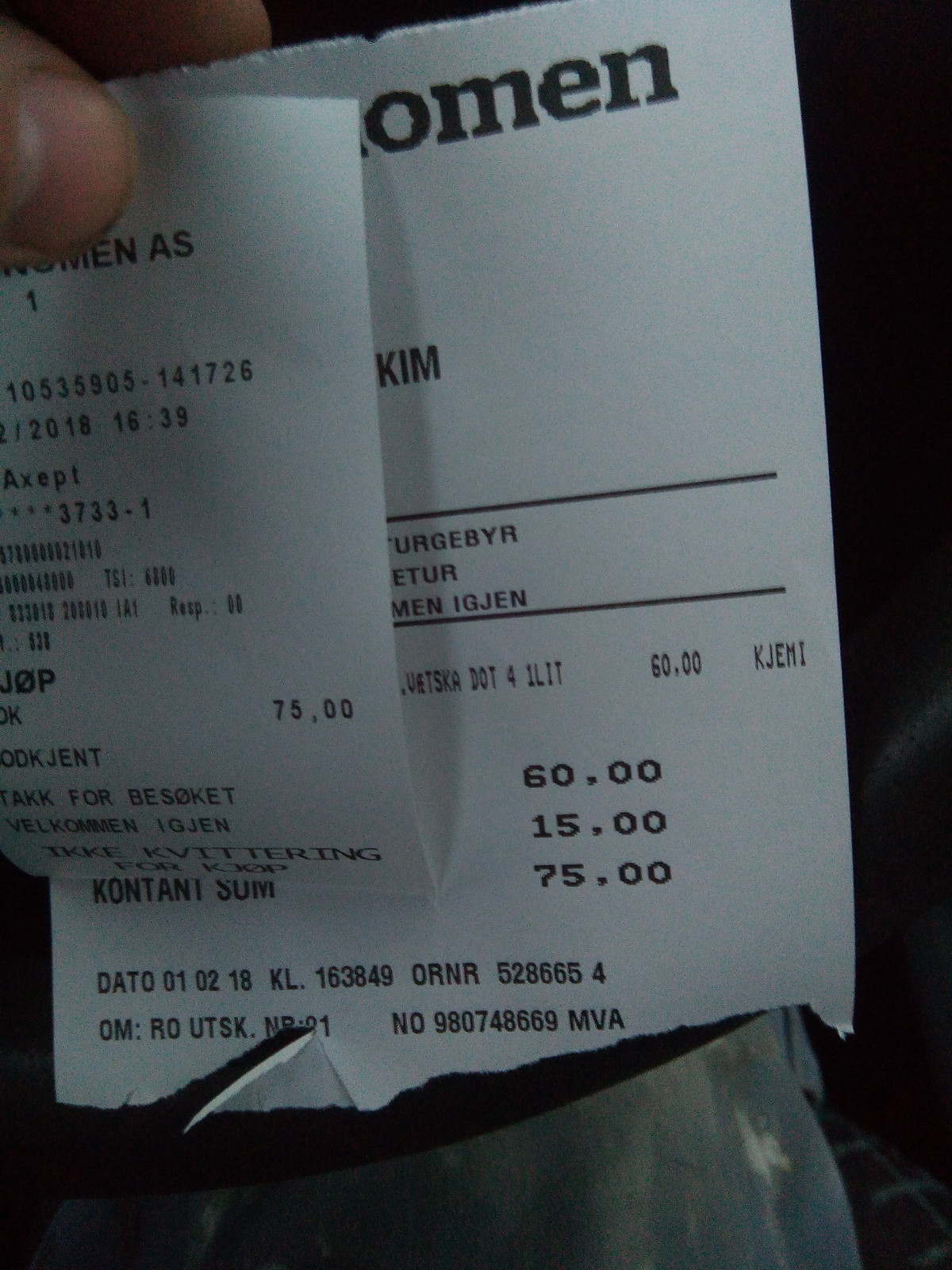In this photo, a person is holding up two small receipts vertically. The front receipt is a tiny, rectangular piece of paper. The tip of the person's thumb is visible in the top left corner of the image, pinching the receipt. Behind it, you can see the index finger supporting a second receipt. The front receipt shows a legible amount of $75. The back receipt has bold black letters at the top and prominently displays the name "Kim" in the middle. This second receipt lists item costs of $60, $15, and $75. In the background at the bottom of the photo, a person is partially visible, wearing grey pants and a black t-shirt.